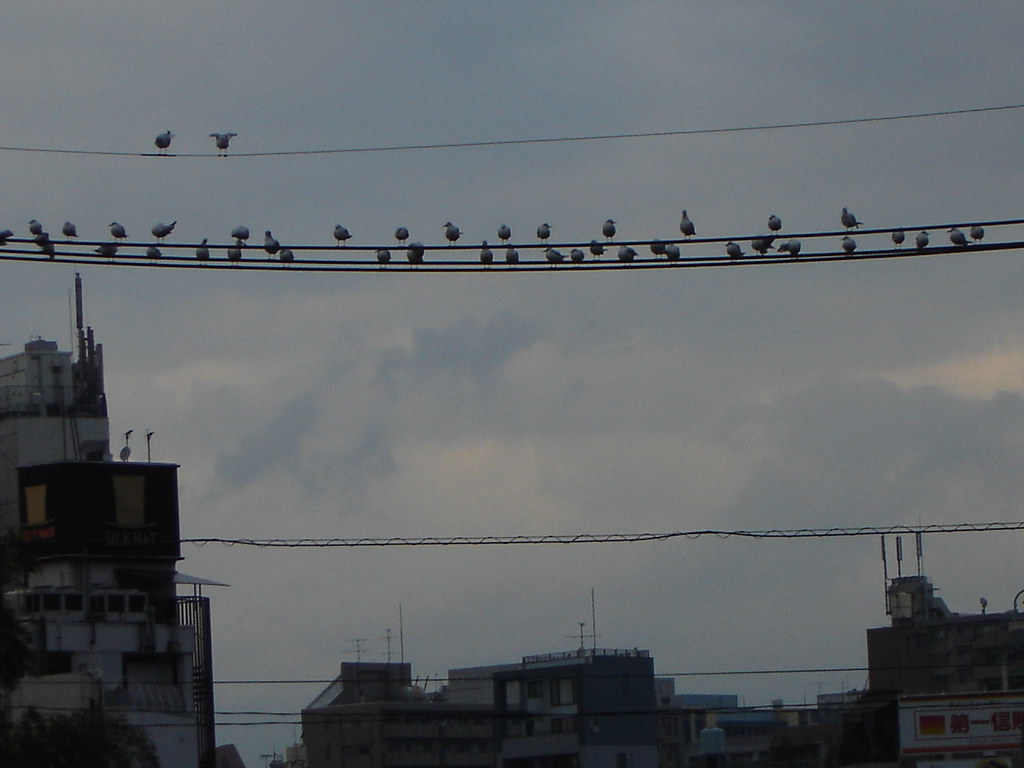This color photograph captures a somber urban scene with muted and dark tones, reflecting an overcast and potentially rainy day. The backdrop features a skyline of industrial buildings, including warehouses, factories, and possibly high-rise apartment structures. The sky is heavily clouded, contributing to the overall gray and depressing atmosphere. Prominent in the photograph are numerous horizontal electrical and telephone wires spanning from left to right across the upper third of the image. These wires host a variety of birds, their silhouettes stark against the gloomy sky. The uppermost wire holds two birds, one seemingly in the act of taking off with its wings slightly outspread. Below, the additional wires are densely populated with up to fifty birds, resting or preparing to take flight. The buildings in the scene are adorned with television antennas, and there is a barely discernible sign above one of the darker structures on the lower right. The overall scene captures a still moment in a dreary, industrial cityscape, dominated by the interplay of silhouetted birds and stark utility lines against a backdrop of foreboding clouds.